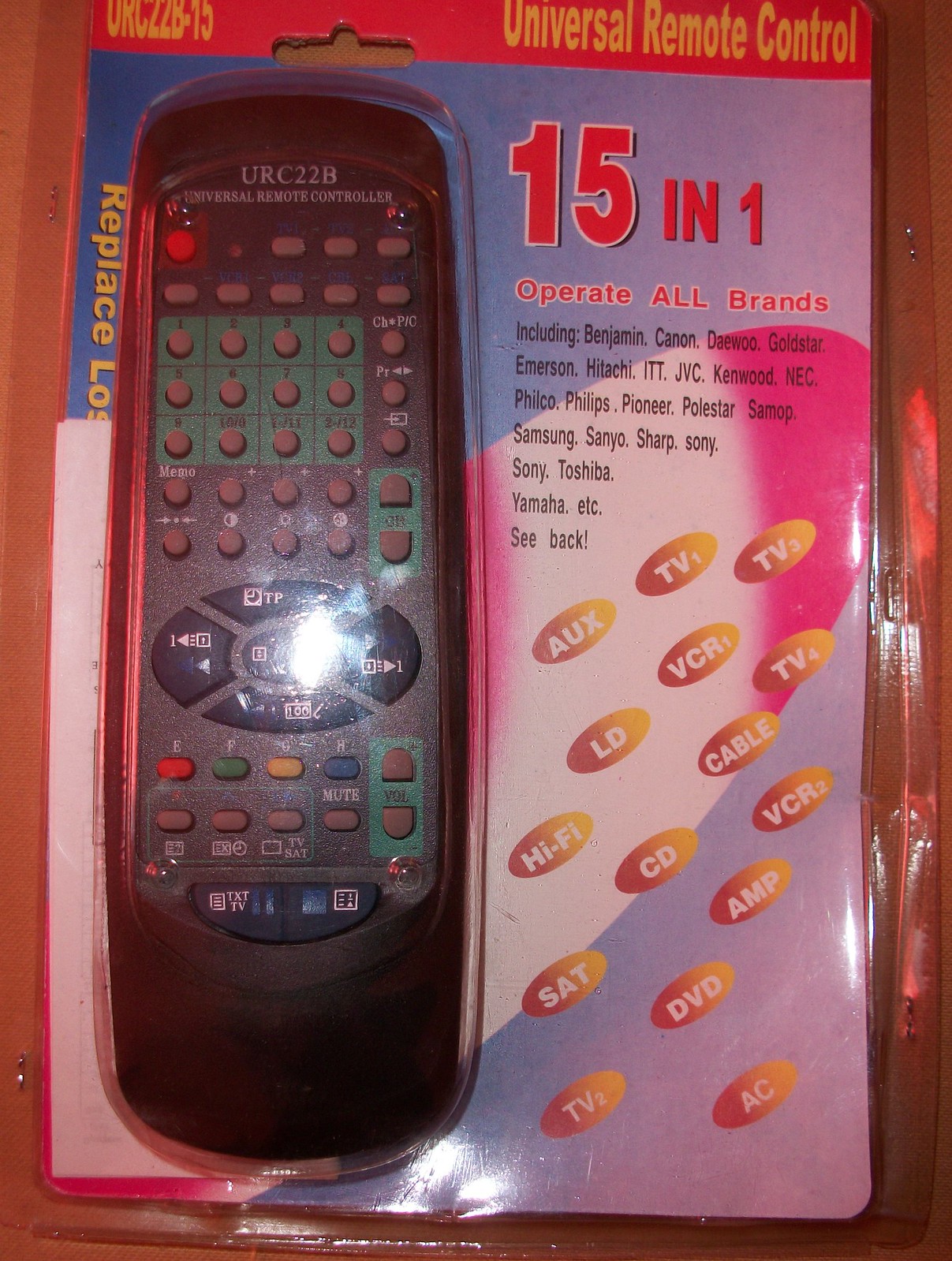This is a detailed digital photograph of a Universal Remote Control, model URC-22B, still in its vibrant, multi-colored packaging. The package prominently features a bright red top with yellow lettering stating "URC22B-15" on the left and "Universal Remote Control" on the right. The background transitions from blue to purple and white, creating an eye-catching effect. The left side of the package has partially readable yellow font text suggesting it replaces lost remotes, while the right side boasts a bold red "15-in-1" claim, emphasizing its capability to operate all brands. The remote is compatible with brands such as Benjamin, Canon, Daewoo, Goldstar, Emerson, Hitachi, ITT, JVC, Kenwood, NEC, Philco, Philips, Pioneer, Polestar, Samsung, Sanyo, Sharp, Sony, Toshiba, Yamaha, among others. It also lists supported devices, including TV-1, TV-2, TV-3, TV-4, VCR-1, VCR-2, VCR-3, LD, Cable, Hi-Fi, CD, Amp, Satellite, DVD, and even AC. Encased in clear plastic, the black remote features around 30 buttons, colored in red, yellow, blue, green, and gray for ease of use. The entire item rests on what appears to be an orangish-colored wooden table. For further details, the package directs to visit www.UniversalTelevision.com.